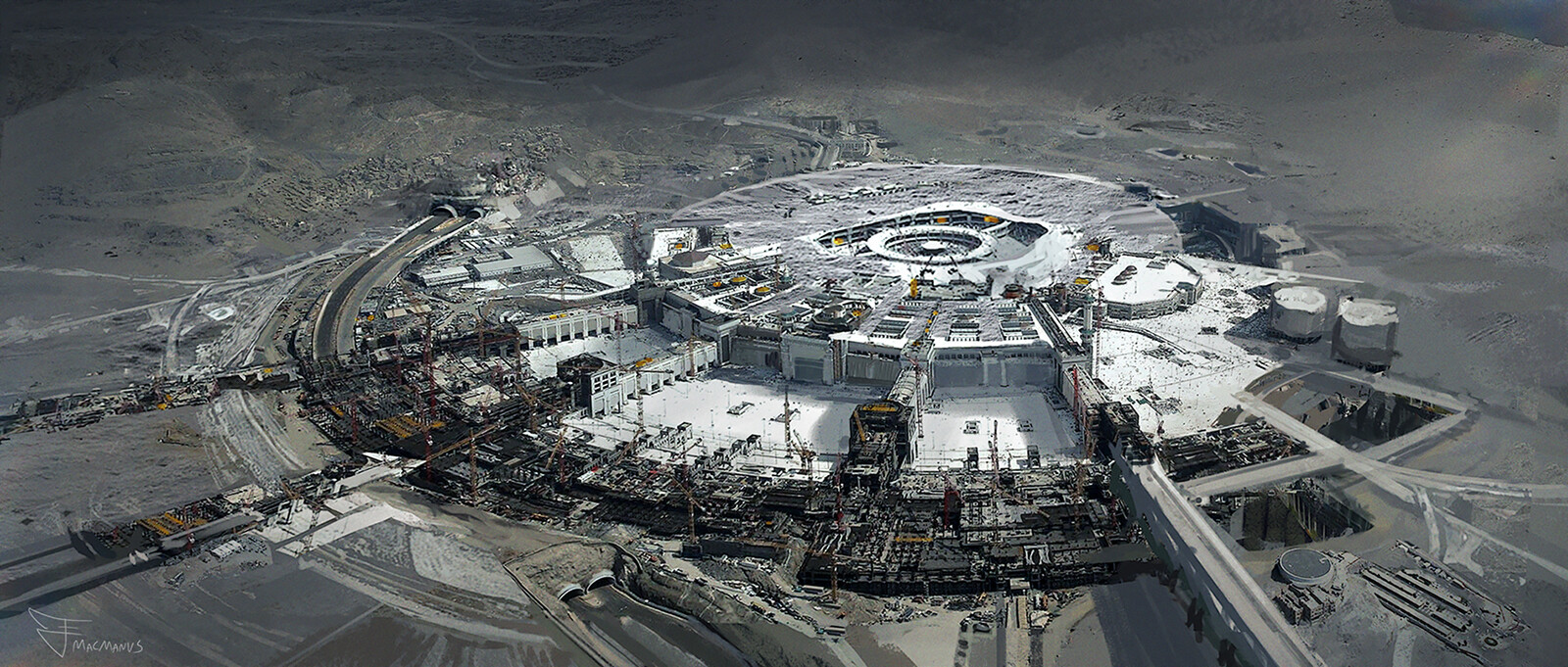The image presents a detailed 3D rendering of a large, round facility that dominates the center, evoking the appearance of an off-world base, possibly on a moon or another planet. This structure is highly futuristic, with a central building that is round and contains a large cylinder in its middle. Surrounding the central area, there are four protruding arms outfitted with numerous cranes resembling those found on the tops of skyscrapers. The cranes form a darker ring around these arms, indicative of a potential mining facility or a large-scale industrial operation.

The overall color palette of the rendering is predominantly gray, with prominent white highlights in the center, enhancing the desolate and stark ambiance of the scene. The ground surrounding the facility is a gray, sandy expanse, adding to the extraterrestrial impression. The rectangular shape of the image reinforces the structured, industrial feel of the environment. The outer edge of the image features a road-like structure, also in gray, which serves as a boundary to the facility.

Despite its industrial and somewhat ominous appearance, with elements that suggest a nuclear power plant or even a deconstructed flying saucer, the precision and scale reflect a setting that is both expensively constructed and potentially hazardous, augmenting the overall otherworldly and unsettling atmosphere of the scene.